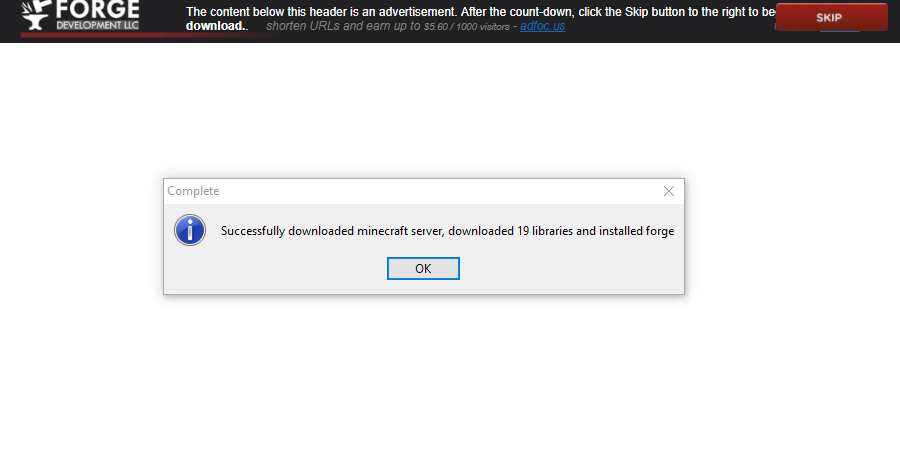The image displays a web page featuring the Forge Development LLC logo located in the top left corner. Adjacent to the logo, there is a text indicating that the content below the header is an advertisement. It instructs the user to wait for a countdown to finish and then click the "skip" button on the right to proceed with downloading. The page advertises earning up to $5.60 for every 1,000 visitors by shortening URLs. A notification appears in the center of the screen, stating that the Minecraft server has been successfully downloaded, including 19 libraries, and Forge has been installed.